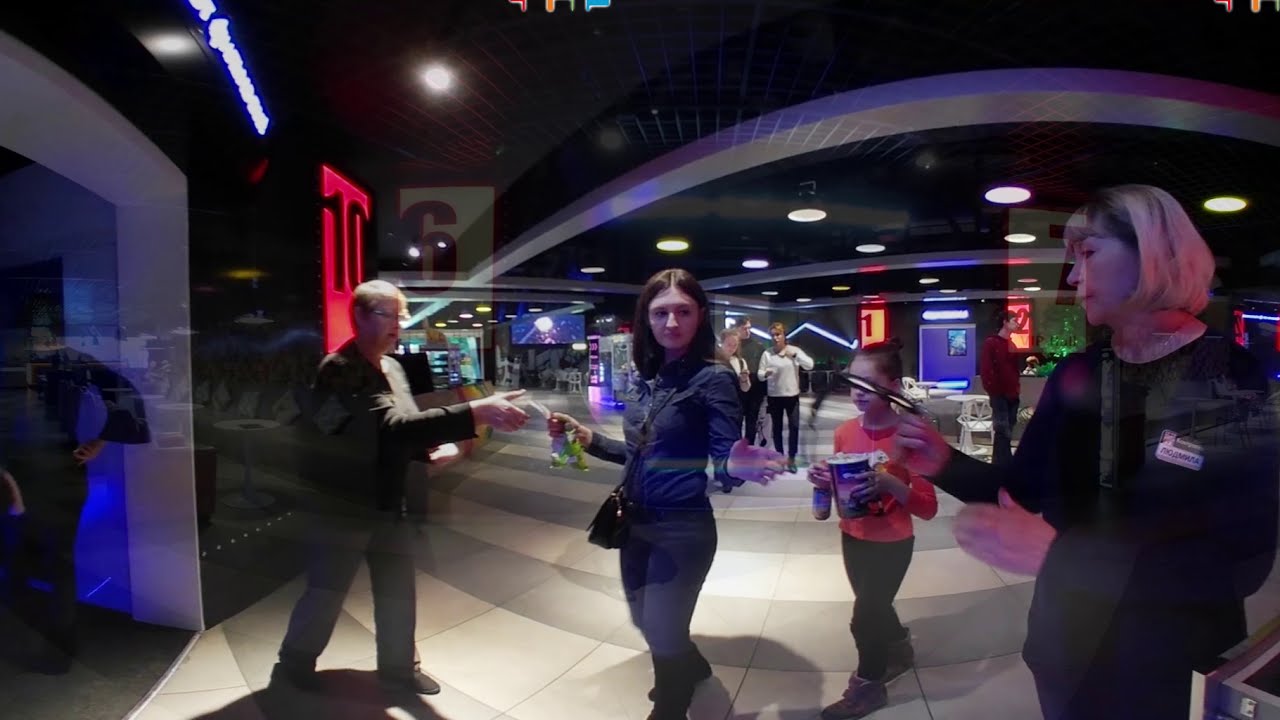The image depicts the inside of a cinema with a dark, thematic ambiance, featuring predominantly black walls and a black ceiling. The floor is composed of white and gray square tiles, creating a contrasting, multicolored pattern. The lighting is recessed, adding to the intense atmosphere, with hints of neon lights enhancing the scene. 

In the foreground, on the right side, a woman in her 50s with short blonde hair is shown examining something in her hand, which is obscured. She wears dark clothing and a name tag. Beside her is a young boy, also dressed in dark clothes, holding a popcorn container. He is Caucasian, with dark, short hair, and wears high-top shoes.

In the center, another woman, with shoulder-length dark hair, dressed in a dark shirt, pants, and shoes, is handing something, possibly a ticket, to a man in long sleeves and blue jeans. The woman has a purse slung over her shoulder. 

Behind them, the image reveals numbered doorways, such as a 10 and a 6, indicating different cinema rooms. The setting is busy, with several people in the distance, further suggesting a bustling family-friendly attraction.